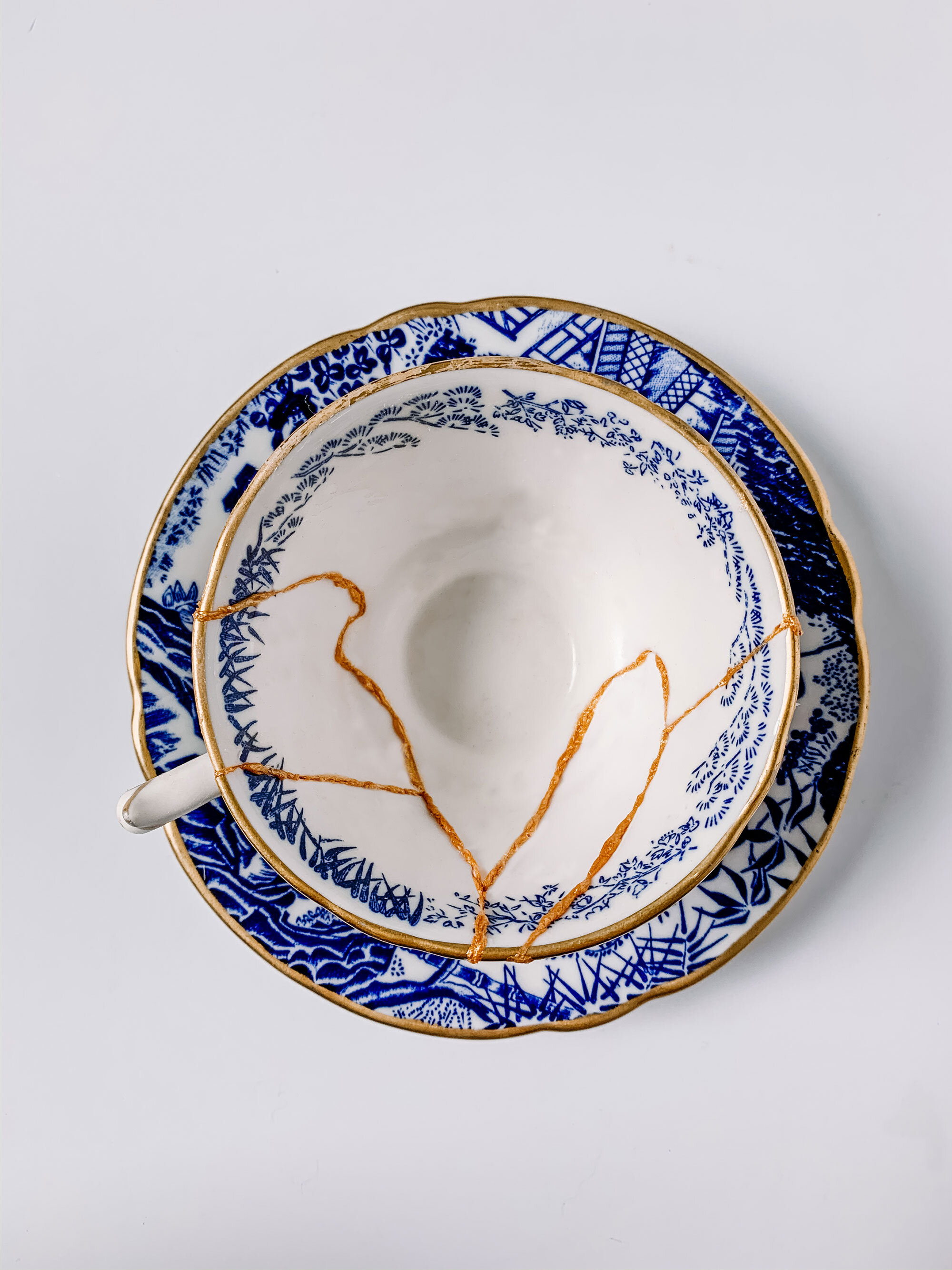The photograph captures a delicate porcelain bowl from a top-down perspective, placed on a light gray, flat surface. The bowl, predominantly white, features intricate blue floral and plant patterns adorning its inner rim. Both the outer and inner rims are elegantly highlighted with gold. Notably, the bowl exhibits signs of having been repaired using the Japanese kintsugi technique, where the fractures have been meticulously mended with gold, creating zigzagged lines that enhance its beauty and history. Adding to the intricacy, a white tab is visible on the bottom left corner of the bowl. The artwork evokes imagery of bamboo and leaves, extending a sense of continuity and charm. Though it isn't explicit in the text, it can be inferred that the bowl may rest on a similarly adorned saucer or plate beneath it, embellished with matching blue and gold patterns.